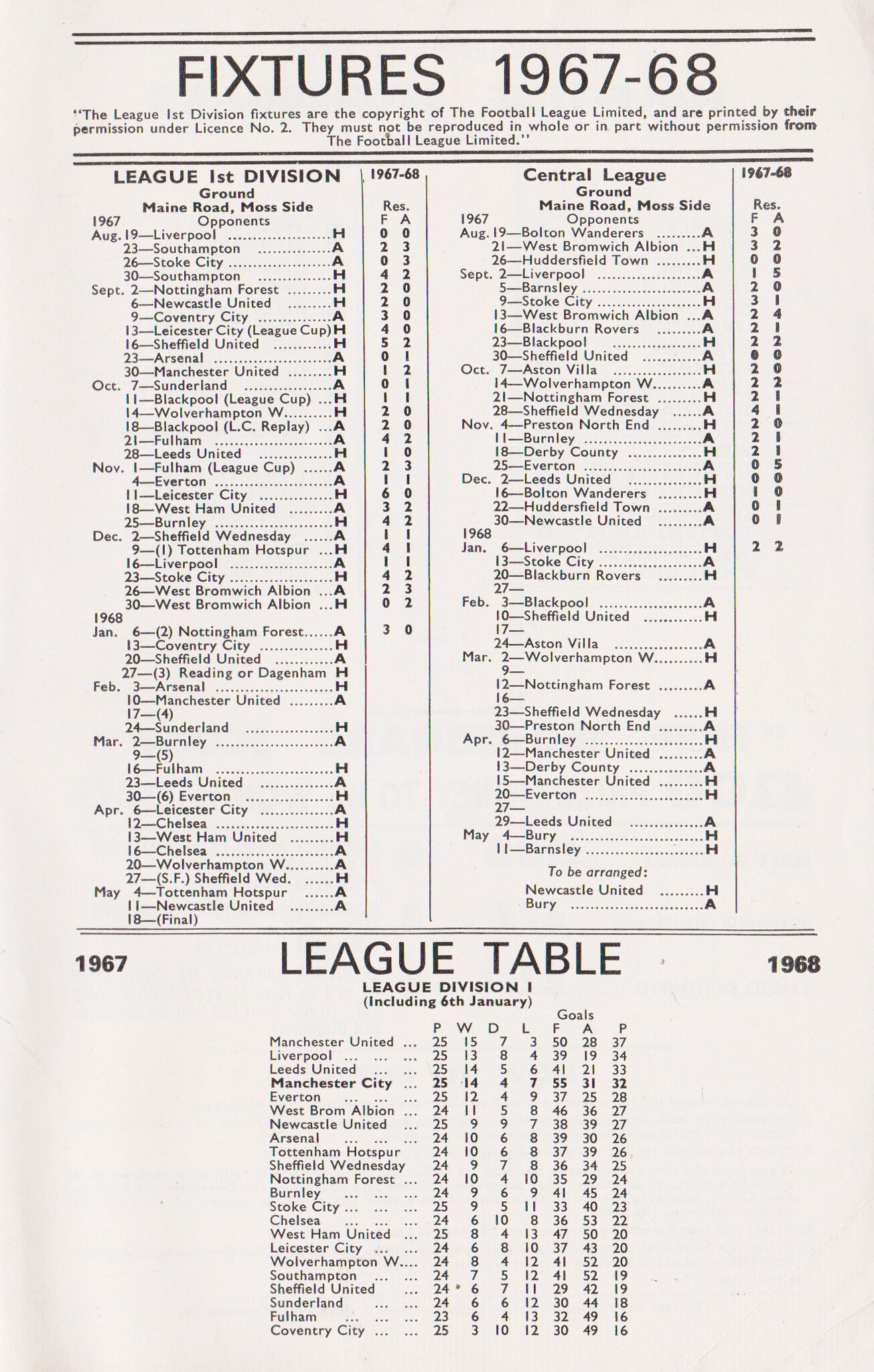The image depicts a detailed pamphlet titled "Fixtures 1967-68" outlining the league fixtures for the First Division, copyrighted by the Football League Limited and printed with their permission under license number 2. Reproduction in whole or in part is prohibited without prior consent from the Football League Limited. At the top section of the pamphlet, there's a structured table listing dates and matches, indicating whether the games will be home (H) or away (A). The fixtures cover the period from August 1967 to May 1968. 

On the left-hand side, it specifies the League First Division Ground at Main Road, Moss Side, with scheduled matches and corresponding home and away statuses. The right-hand side mirrors this information for the Central League Ground, Main Road, Moss Side, similarly detailing the games from August to May. 

At the bottom of the pamphlet, there's a league table with the title "League Division 1," featuring team names as of the 6th of January. Included prominently are teams like Manchester United and Liverpool, alongside the comprehensive schedule for the league season of 1967-1968.